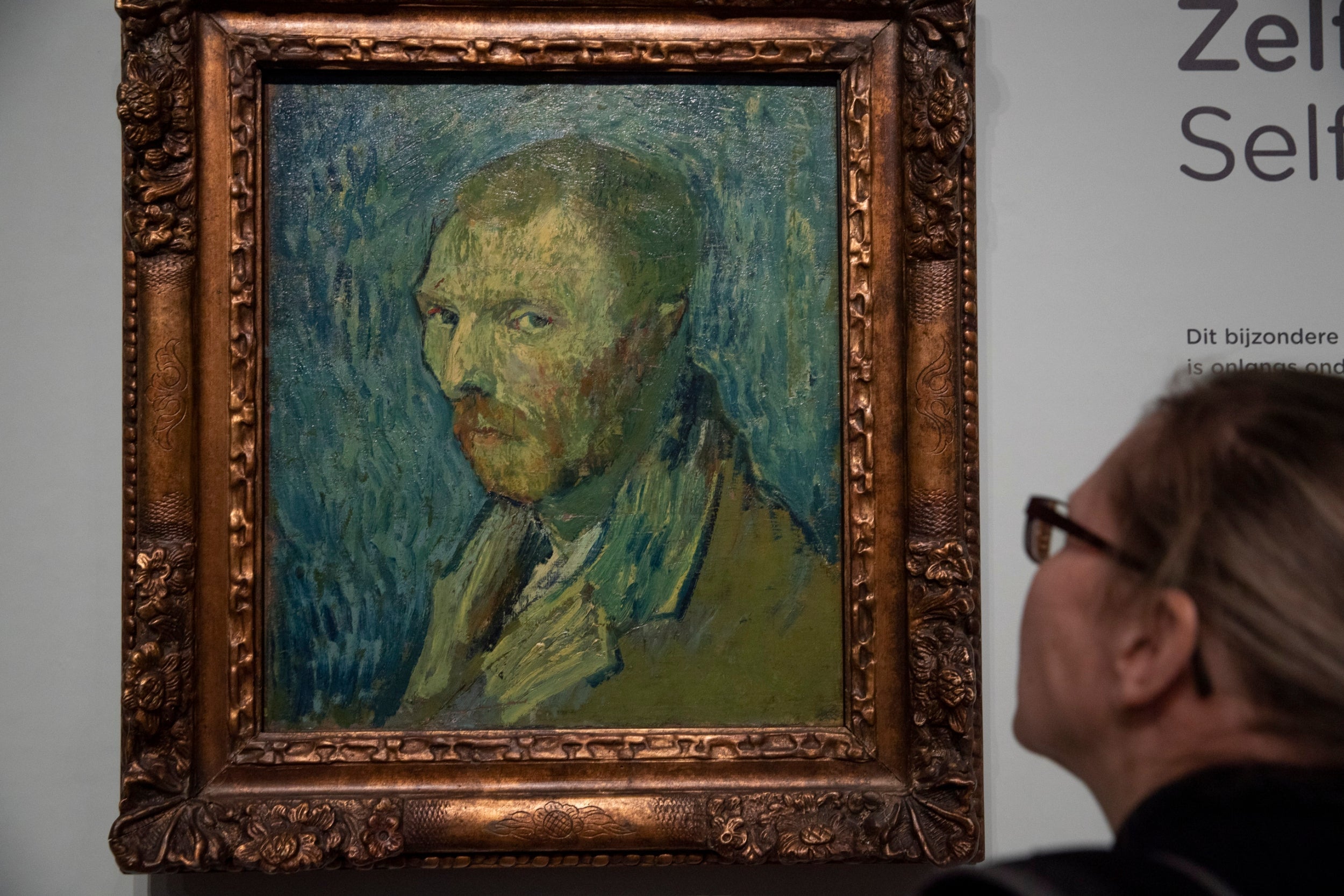The horizontally aligned image captures a close-up scene of a woman in glasses with her brown hair pulled back, observing an old painting indoors. Positioned in the lower right corner, the left side of her face is visible from slightly behind and in profile. The subject of her attention is a framed oil painting, prominently featuring Vincent van Gogh in an ornate, copper-detailed, thick metal frame with a brownish hue. Van Gogh’s self-portrait showcases his upper body, focusing on his face and the left side of his shoulder, clad in a brownish-green collared jacket. He has a brown mustache, slightly discontented expression, and blue eyes set against a background of wavy blue lines in varying shades. The surrounding wall, a light gray color, features partial text in the upper right corner, with visible letters "Z-E-L-T" and "S-E-L-F" before being cut off. Above Van Gogh’s head, smaller text reads "Dit bijonder," suggesting the inscription may be in Dutch. The overall composition, despite the slightly blurry capture of the woman, conveys a deliberate moment of contemplation and connection with the iconic artwork.